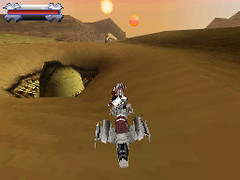This image depicts a pixelated screenshot from an older video game, set in a desert landscape under an orange and pink sky. The scene is rendered in poor quality, emphasizing its vintage nature. In the upper left-hand corner, there's a rectangular health bar with a thin red line running through the middle, overlaying shades of light and dark colors.

The main setting features undulating sand dunes and jagged cliffs in the background. The bleak desert ground appears dry and brown. The sky, dominated by a sunset, shows a mix of light pink and orange hues. Positioned towards the top center of the sky, there's a circular fireball-like object, entirely orange, possibly representing a celestial body, and another round circle lower to its right, which could be a setting sun.

Central to the image is a gray spaceship with wings, moving forward into the desert. The spaceship is primarily silver, detailed with black on its tail and maroon on its body. Notably, in front of the spaceship on the left side of the image, a crater with a lighter-colored dome rising out of it can be observed, adding to the barren, alien-like environment.